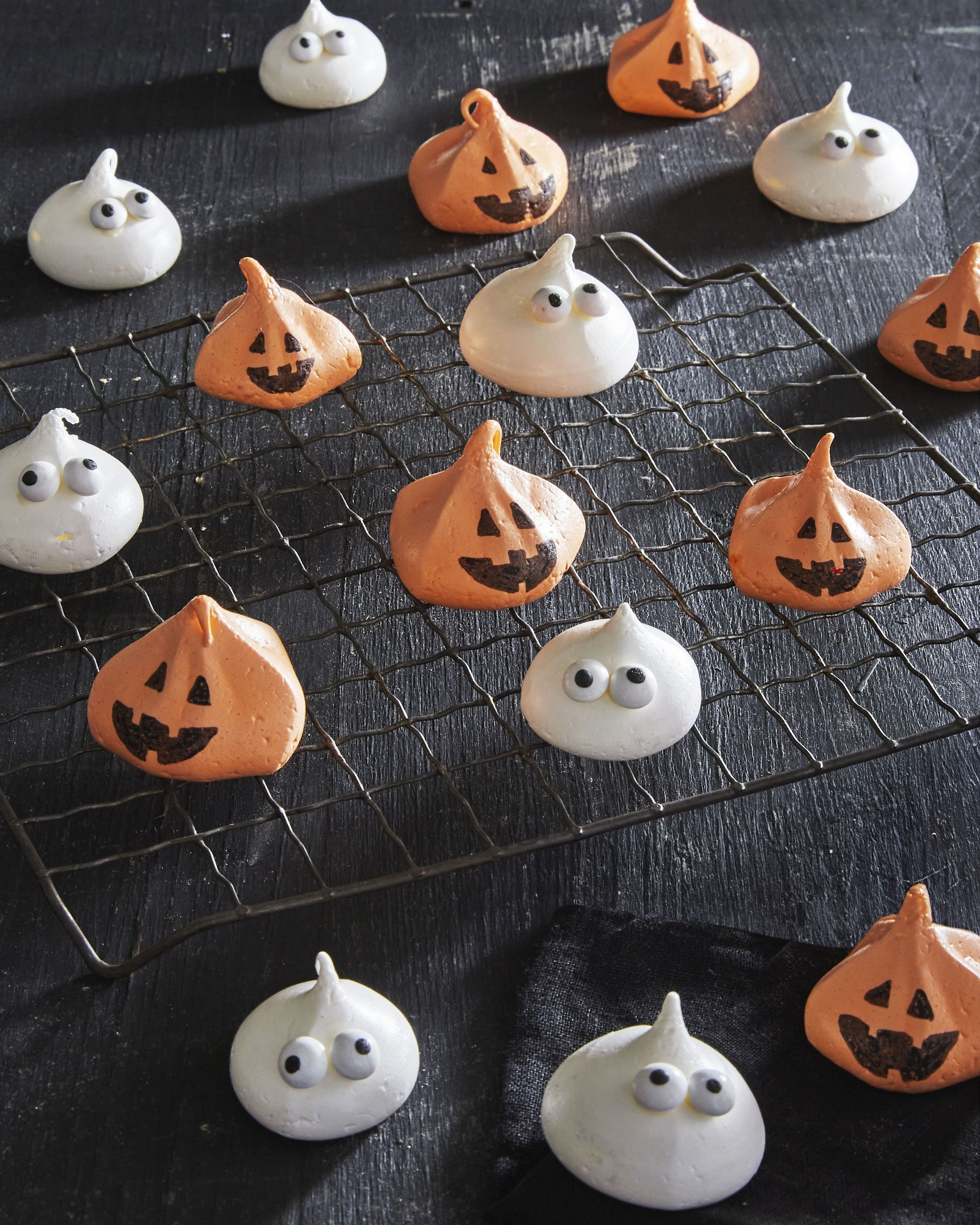This color photograph features a wire rack positioned diagonally from left to right in the center of the image, showcasing a delightful assortment of Halloween-themed meringue cookies. There are seven cookies displayed on top of the rack, with an additional three placed directly in front of it and six more scattered behind, adding a playful and festive atmosphere. Illuminated by a light source from the right, the cookies are vividly highlighted against the black, textured wooden backdrop, which beautifully enhances their vibrant hues and forms.

The cookies include two distinct designs. The first design comprises orange meringues with twisted tops, each meticulously decorated with a jack-o'-lantern face, adding a whimsical touch. The second design features ghost-shaped meringues, characterized by their flat, blob-like base and pointed tip, complete with adorable googly eyes that appear to be crafted from candy decorations.

The meticulous detail in the photograph captures the light reflecting off the meringues, emphasizing their airy, fluffy consistency. The surface texture of the cookies reveals tiny pores, further indicating their light and spongy nature. Overall, the image eloquently portrays the playful spirit of Halloween through these intricately crafted treats, set against a rich, textured background.